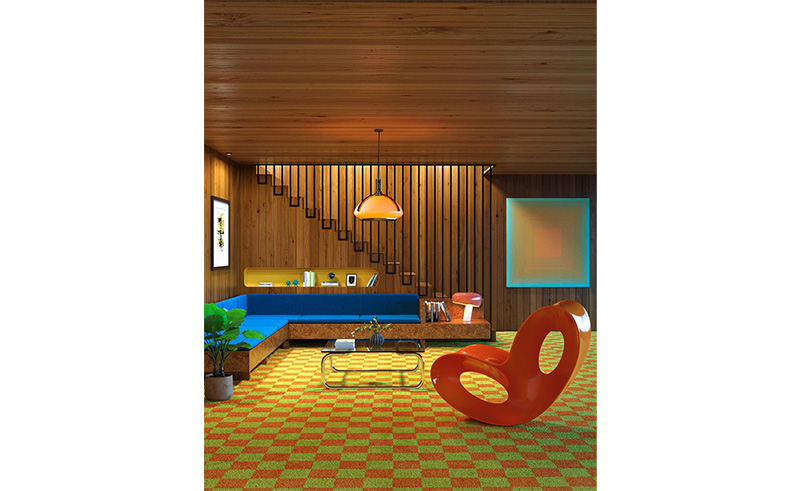The image captures a room with a unique blend of 1970s retro and modern contemporary decor. The walls and ceiling are entirely paneled with medium brown wood, evoking a nostalgic yet stylish atmosphere. Dominating the room is an L-shaped couch with a wooden base and royal blue cushions, accompanied by a matching brown wooden end table featuring a distinctive mushroom-shaped lamp. In front of the couch is a sleek, modern glass coffee table adorned with a plant and some knickknacks.

To the left of the couch, a large floor plant adds a touch of greenery, while a bright red, shiny plastic chair with a mask-like design stands out as a bold accent piece. Nearby, a small glass table with silver legs also supports a plant and a book. The checkered carpet, composed of alternating red and green squares, covers the entire floor, enhancing the room's vibrant color scheme.

Behind the couch, there is a built-in cubby within the wall of the stairs, filled with various books and photographs. The wall on the left features stairs ascending, while the right side displays a large piece of modern art with a blue frame surrounding an orangey-pink center. Another artwork, a white picture with yellow and black in the center, can be spotted on the left wall.

A modern, globe-like chandelier with a gold finish hangs from the ceiling, casting a warm glow over the eclectic and carefully curated decor.